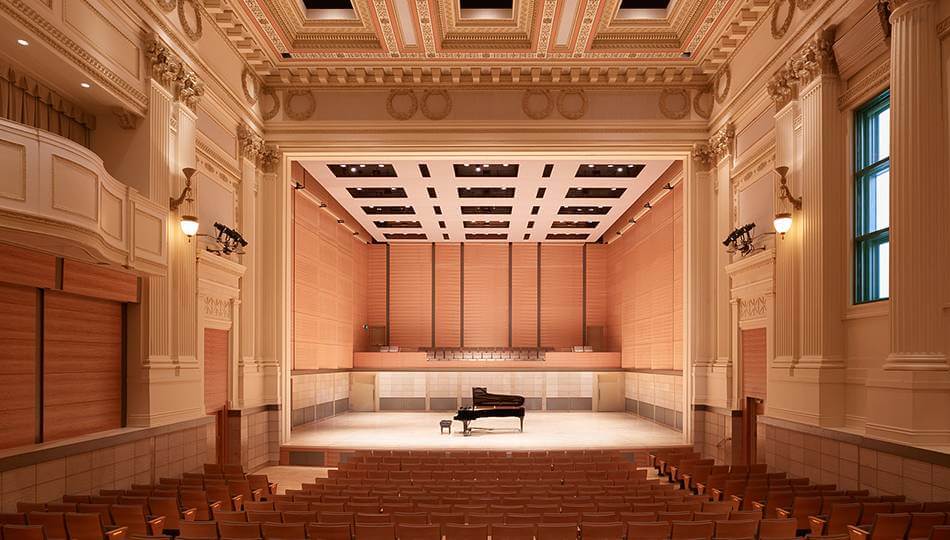This image captures a beautiful, empty concert hall taken from the back of the auditorium, showcasing rows of unoccupied seats leading down to a stage. The color scheme features elegant tones of white and medium wood, with an ornate coffered ceiling adding grandeur to the setting. The seats are arranged centrally with aisles on both sides, and additional seating extends from these aisles. Dominating the stage is a grand piano made of dark wood, positioned under stage lights that shine against a black backdrop. A window on the upper right allows natural light to filter in, while to the left, a balcony section with exclusive seating offers a more private view. The interior's design has a refined, Renaissance-inspired aesthetic, complementing the hall's sophisticated atmosphere.